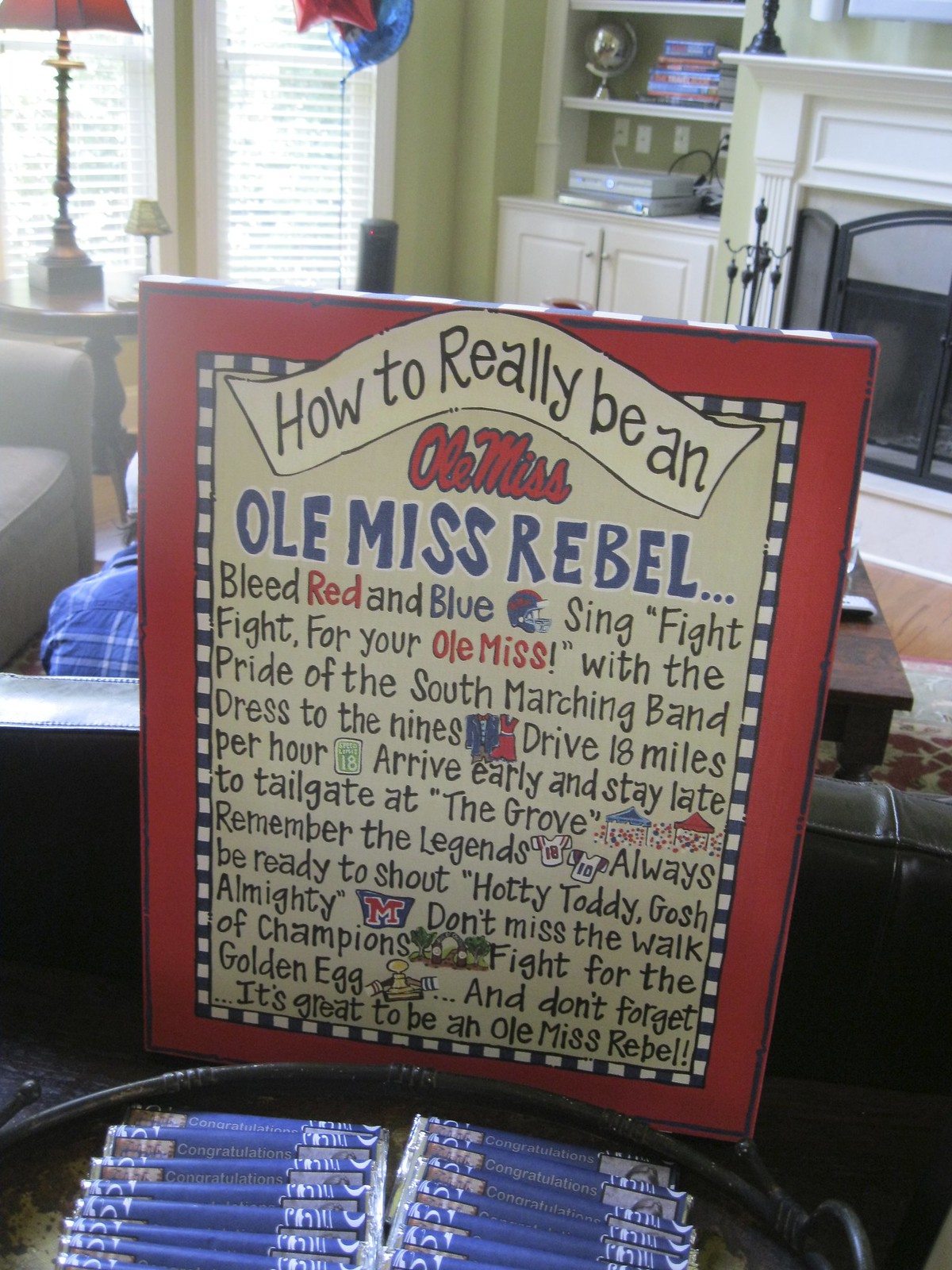This image depicts a brightly lit indoor living room with sunlight streaming through windows adorned with horizontal blinds on the left. A red lamp with a red lampshade sits on a table by these windows. The focal point of the photograph is a prominently displayed handcrafted sign, propped up against the back of a couch. The sign features a red border with blue and black lettering and states: “How to really be an Ole Miss. Ole Miss Rebel. Bleed red and blue, sing Fight, Fight for your Ole Miss with the Pride of the South marching band, dress to the nines, drive 18 miles per hour, arrive early and stay late to tailgate at the Grove, remember the legends, always be ready to shout, Hotty Toddy, Gosh Almighty, don’t miss the Walk of Champions, fight for the golden egg, and don't forget it's great to be an Ole Miss Rebel.” In front of the sign is a plate filled with candy bars that say "congratulations." To the right, there is a white fireplace with a black door, and nearby, white furniture can be seen. Also visible is the back of a man's head, adding a human element to the cozy and fan-spirited setting.